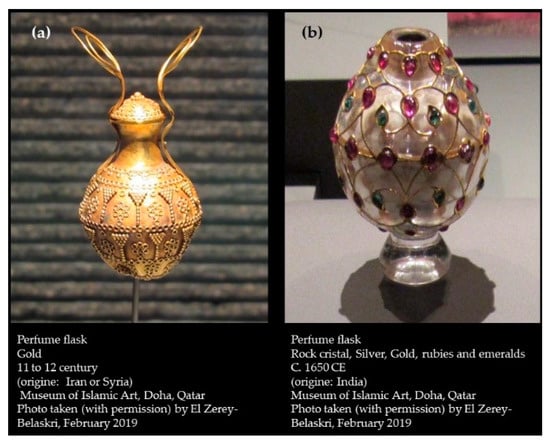The image features two historical perfume flasks, likely sourced from an auction catalog or an educational reference such as a history or art textbook. The left flask, labeled as Perfume Flask A, dates back to the 11th to 12th century and is crafted from gold. Originating from Iran or Syria, it is housed in the Museum of Islamic Art, Doha, Qatar. The photograph, taken by Elzeri Belaskri in February 2019, depicts a small, intricately designed gold flask with a rich golden hue, adorned with engravings and symmetrical patterns resembling martini glasses. The flask features handle-like structures near the top.

Perfume Flask B, on the right, is a luxurious piece dating to circa 1650 CE and is adorned with rock crystal, silver, gold, rubies, and emeralds. Originating from India, it is also part of the collection at the Museum of Islamic Art, taken by the same photographer and during the same period as the left flask. The flask has a pearly base with a layer of clear crystal over it, embellished with opulent gold filigree and studded with colorful gemstones. Both flasks are noted for their rich and elaborate designs, showcasing historical craftsmanship and luxury.